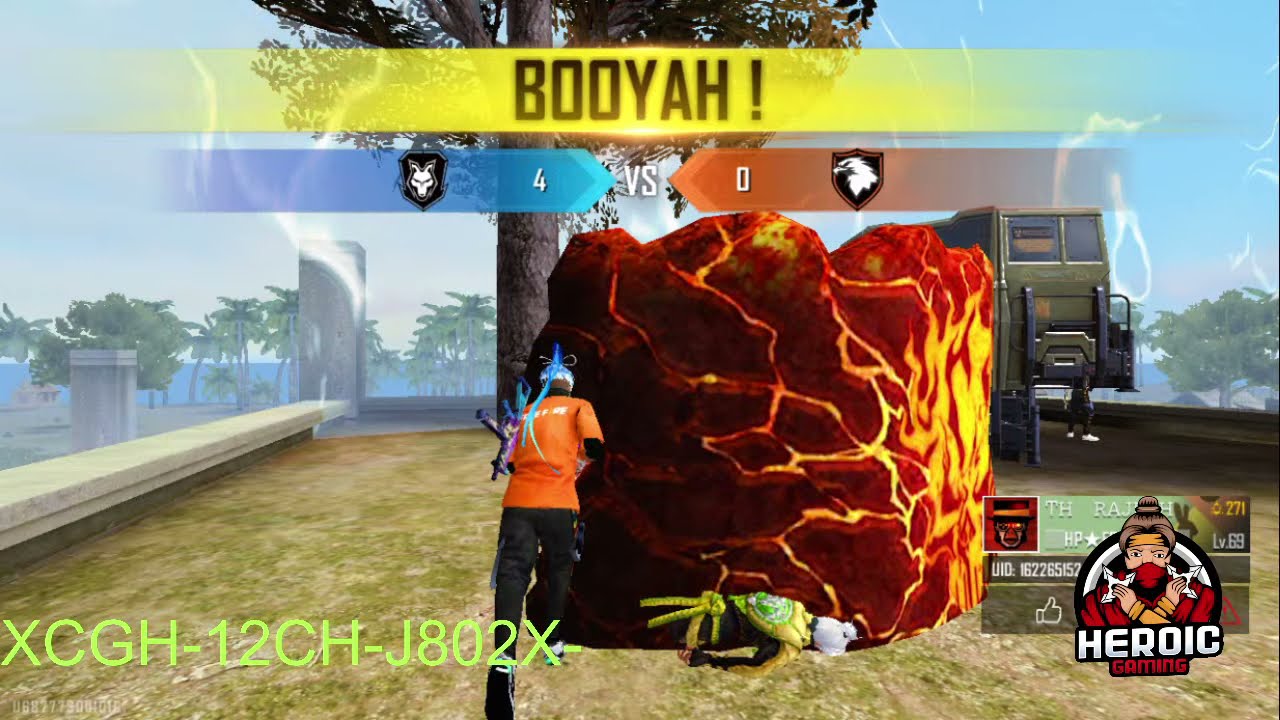The screenshot captures an intense moment from a video game, featuring a character in an orange shirt and black pants sprinting towards a massive block of molten lava, glowing intensely in red, yellow, and orange hues, creating a visually striking scene. At the top of the screen, bold yellow and black text exclaims "Booyah!" with an exclamation point, indicating a significant achievement or victory. On the left side of the screen, a blue tab displays the number four alongside an icon resembling a character or bug, while on the right, an eagle icon accompanies the number zero, possibly representing a score or status indicator. The background reveals a diverse landscape with trees and a truck situated on what appears to be a rooftop, suggesting a dynamic environment that could be part of a game similar to Fortnite, complete with a visible shrinking shield area. In the lower right corner, the text "Heroic Gaming" is displayed, along with a gamer tag, indicating the player's identity. The vivid colors—orange, black, blue, green, brown, yellow, and red—add to the immersive and high-stakes atmosphere of the game.